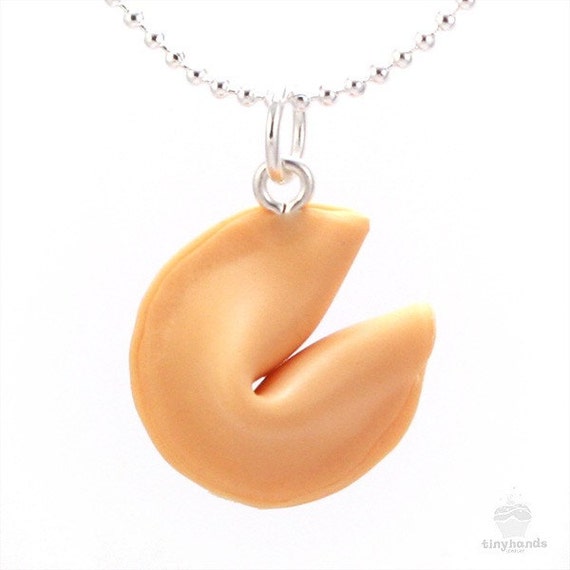This detailed close-up showcases a fortune cookie pendant intricately designed to resemble a real fortune cookie. The light tan pendant, with its realistic folded texture around the edges, is hooked via a small round clasp to a silver beaded necklace. The pendant hangs with the tips of the fortune cookie facing right on a transparent white background. In the bottom right corner of the image, there is a watermarked Tiny Hands logo, depicted as a small, gray emblem that resembles a cupcake, with subtle, light text beneath it. Despite differing opinions on its material quality, the pendant’s shine adds to its visually striking appeal, making it a unique piece of jewelry.